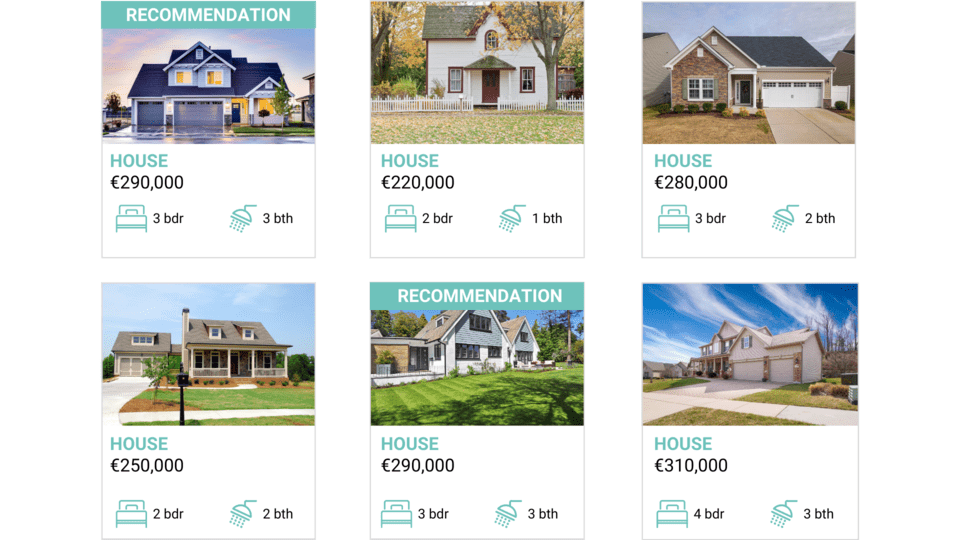The image showcases various advertisements for homes on the real estate market, each with detailed descriptions and pricing. There are six distinct listings, displayed in two rows, arranged from left to right. 

In the top row:
1. The first house, priced at $290,000, features three bedrooms and three bathrooms. This particular listing is prominently recommended, identified by a green bar with white text at the top.
2. Next is a house listed at $220,000, offering two bedrooms and one bathroom.
3. The third house in this row is priced at $280,000 and includes three bedrooms and two bathrooms.

In the bottom row:
1. The first house on the left is listed for $250,000 and features two bedrooms and two bathrooms.
2. Adjacent to it is another $290,000 listing, mirroring the first house with three bedrooms and three bathrooms. It is also a recommended listing, highlighted similarly with a green bar and white text at the top.
3. The final house in this collection is priced at $310,000 and boasts four bedrooms and three bathrooms.

All icons representing the number of bedrooms and bathrooms are displayed in a green-blue color scheme with the accompanying text in black lettering, ensuring clarity and uniformity across the advertisements.